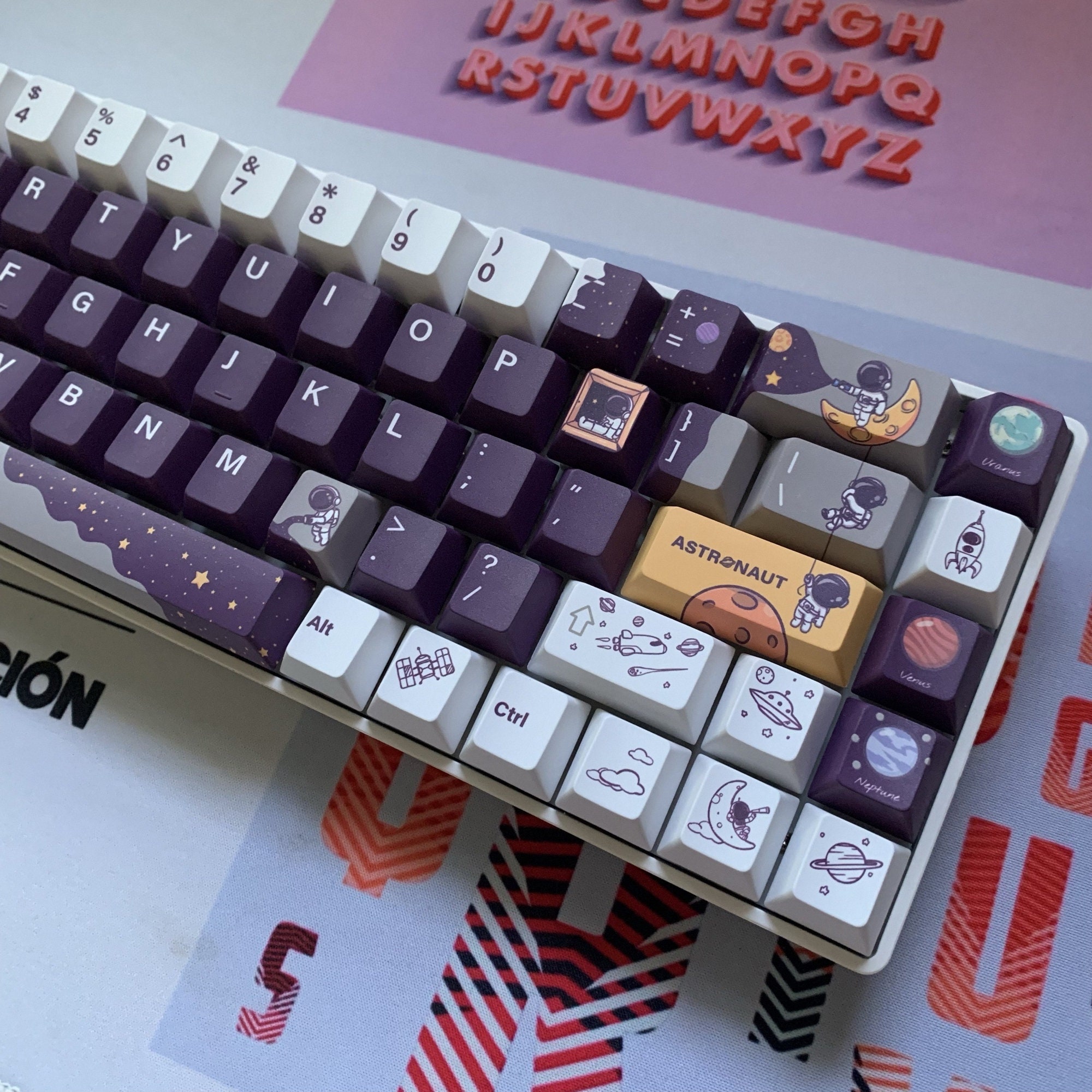The image showcases a uniquely designed keyboard with an astronaut theme placed on a tabletop. The majority of the keys are a dark purple color, while the number keys (four through zero) are a bright white. The enter key features a yellow astronaut along with clip art images of spaceships and a cartoon astronaut. Other keys also display celestial designs: the bracket and backslash keys have astronaut images, the delete key has an astronaut on a moon crescent, and some other keys feature planets and spacecraft, including a depiction of Earth. The space bar is gray, adorned with black portions filled with stars and star-shaped dots. The elevated keys liken it to a gaming keyboard. Below the keyboard, there is a piece of paper with abstract, colorful striped letters. This detailed artwork and thematic stickers add a vibrant and distinctive touch to the keyboard.